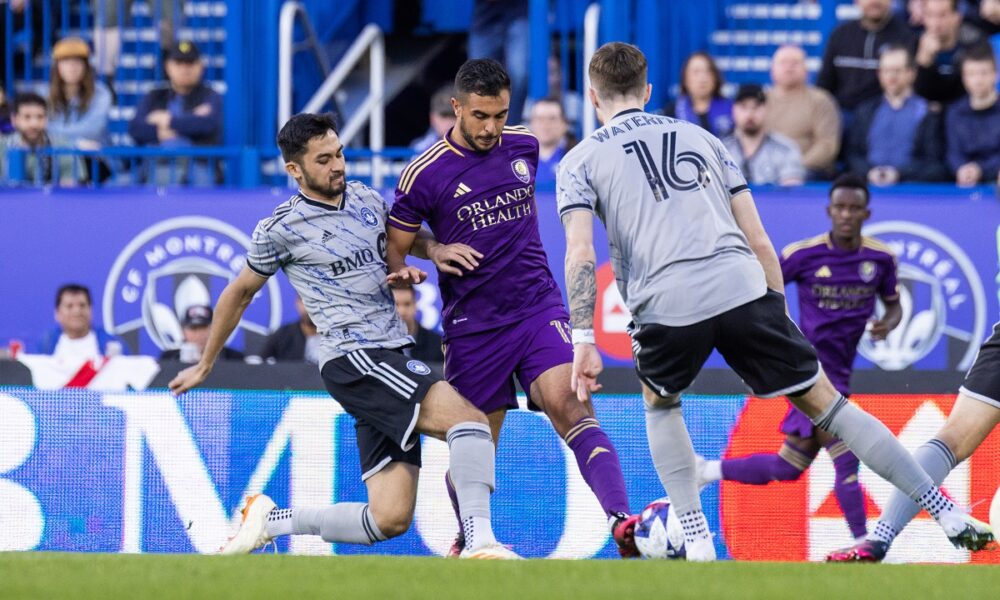In this vibrant soccer match set in an American stadium, four men dominate the field with intense action, reflecting the team spirit and competitive nature of the game. Two players clad in purple jerseys, shorts, and socks from Orlando Health are engaged in a critical play. One of them is poised with his leg bent back, ready to kick the ball, while a player in a gray jersey with black shorts and gray socks is moving in to intercept and block the kick. The other purple-clad teammate runs alongside, closely watching the play unfold. The stands in the background are filled with spectators, seated on blue bleachers, separated from the field by a blue divider. The bleachers display a prominent red and white logo amidst the buzzing ambiance of the stadium. Although the scene is slightly blurry, the energy and intensity of the game are palpable, capturing a moment filled with athleticism and strategic prowess.